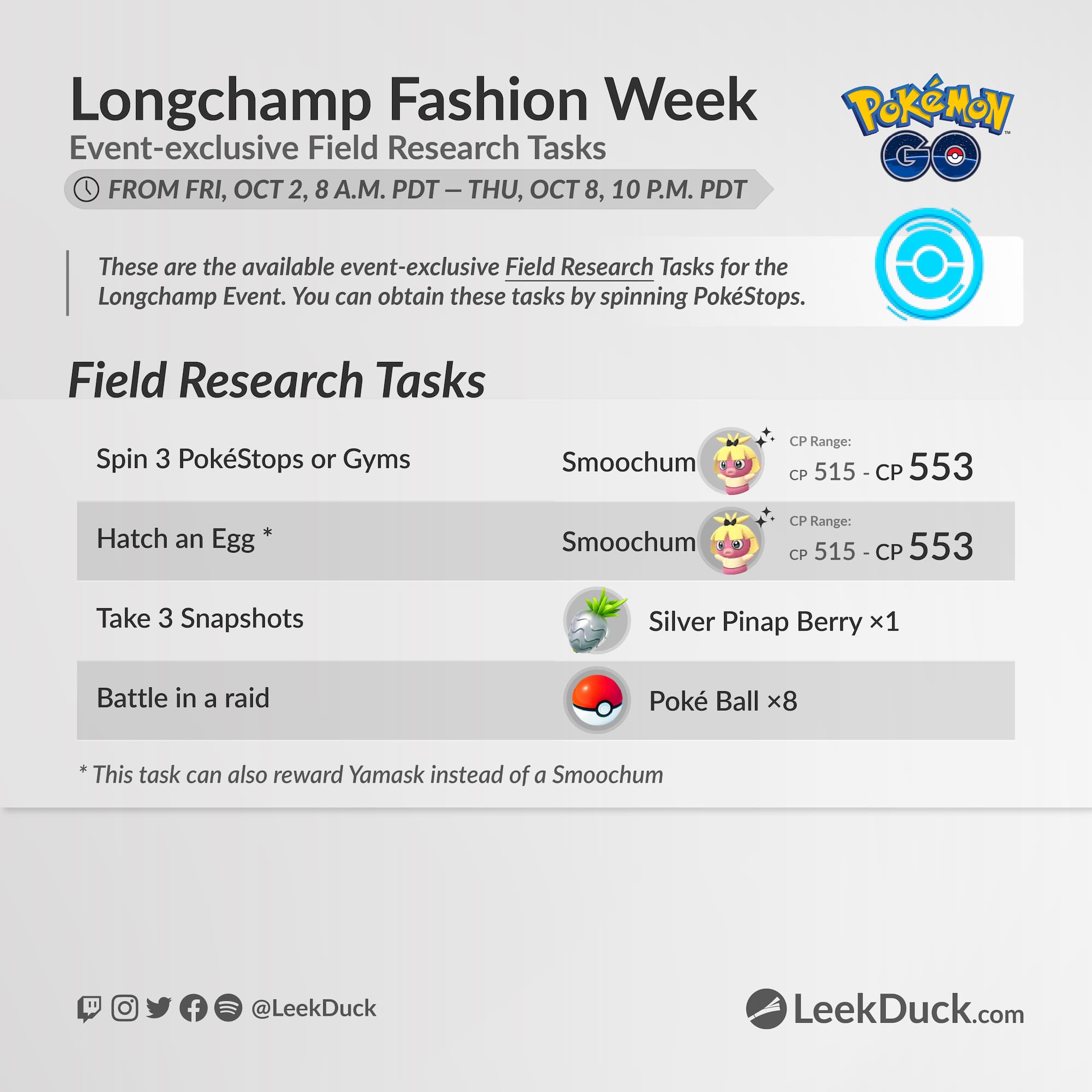Here is a detailed and cleaned-up caption for the screenshot:

---

This screenshot from the website leakduck.com highlights the Pokémon GO Longchamp Fashion Week event. At the top of the page, "Longchamp Fashion Week" is prominently displayed alongside the Pokémon GO logo. Below this, text describes event-exclusive Field Research tasks scheduled from Friday, October 2nd, 8 a.m. PDT to Thursday, October 8th, 10 p.m. PDT. Players can acquire these tasks by spinning PokéStops.

The specific Field Research tasks listed are:

1. Spin three PokéStops or Gyms - Reward: Smoochum (represented by the Smoochum character).
2. Hatch an Egg - Reward: Smoochum.
3. Take three snapshots - Reward: Silver Pinap Berry (displayed with an image of the berry).
4. Battle in a Raid - Reward: Poké Ball (note: this task can also reward Yamask instead of Smoochum).

At the bottom of the page, icons for Instagram, Twitter, Facebook, Spotify, and an unspecified platform are displayed, followed by the handle @LeakDuck.

---